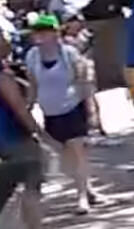A blurry image captures a woman in mid-walk on a sidewalk, potentially leaning on a structure to her right. She is wearing a baseball cap with a bright green crown and a dark-colored bill. Her outfit consists of a white short-sleeved shirt layered over a black undergarment, paired with black shorts. Her long dark hair, possibly styled in braids, cascades down in front of her. The photograph juxtaposes a well-lit background with the shaded area where the woman is positioned, creating a contrast that highlights her figure amidst the softer light.